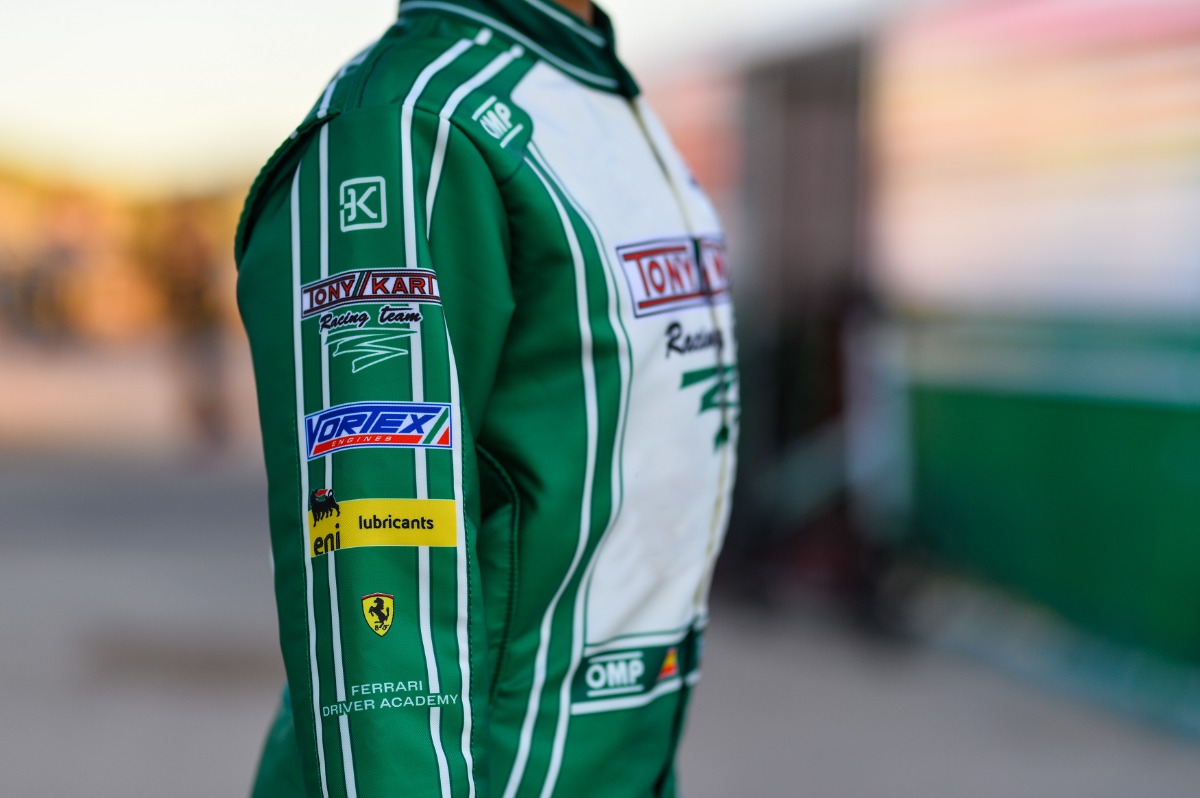The image features a detailed close-up of a go-kart racing suit prominently displayed in the center. The suit, which is primarily green with a white frontal section, includes several distinguishing markings and patches. The front white area displays red text reading "Tony," with the words "Racing Team" prominently beneath in black letters. A signature element is the series of white stripes running down both long green sleeves. One sleeve is adorned with multiple patches: a white square with a letter "K," red lettering that spells "Tony Kart," a blue patch labeled "Vortex," and a distinctive yellow oblong square that says "Lubricants ENI." Additionally, there's an emblem showing a horse and the "Ferrari Driver Academy" branding. The background of the image is blurred, keeping all focus on the intricate details of the racing suit.